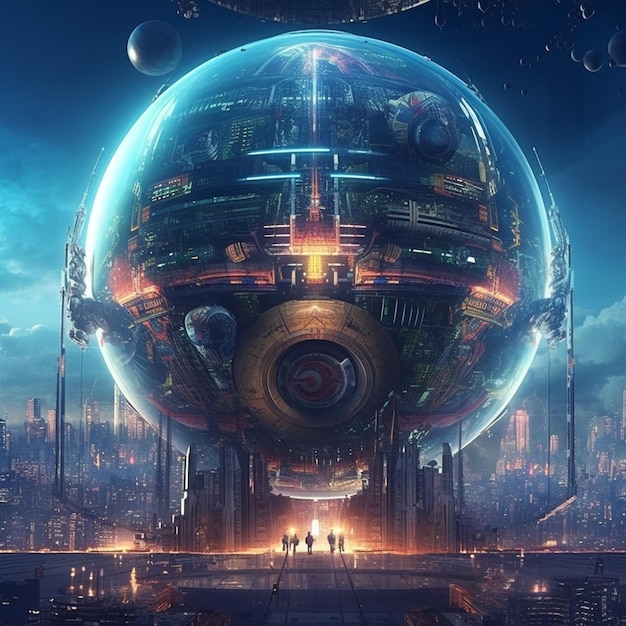This vividly detailed, futuristic image showcases a strikingly modern digital artwork that appears to be computer-generated. Dominated by a large, transparent orb filled with intricate machinery and circuitry, it hovers above a densely populated, brightly lit futuristic cityscape. The orb, evocative of advanced spacecraft seen in sci-fi movies, is illuminated with a spectrum of colors, including blues, grays, yellows, golds, and pinks, adding an extra layer of complexity and wonder.

The background features a dark blue sky merging into the vastness of space, dotted with planets and ethereal orbs. This celestial canvas provides a stark contrast to the sprawling city below, whose skyline is alive with vividly illuminated buildings in fiery reds, oranges, and yellows.

In the middle of this scene, shadowy figures of four to five people can be seen moving either towards or away from the glowing orb, rendered tiny by comparison to the colossal structure above them. This positioning and their movement towards the light give the image an enigmatic and story-like quality, as though capturing a moment from a futuristic film. Overall, the picture is a mesmerizing blend of futuristic science fiction elements and deeply detailed contemporary artistry.